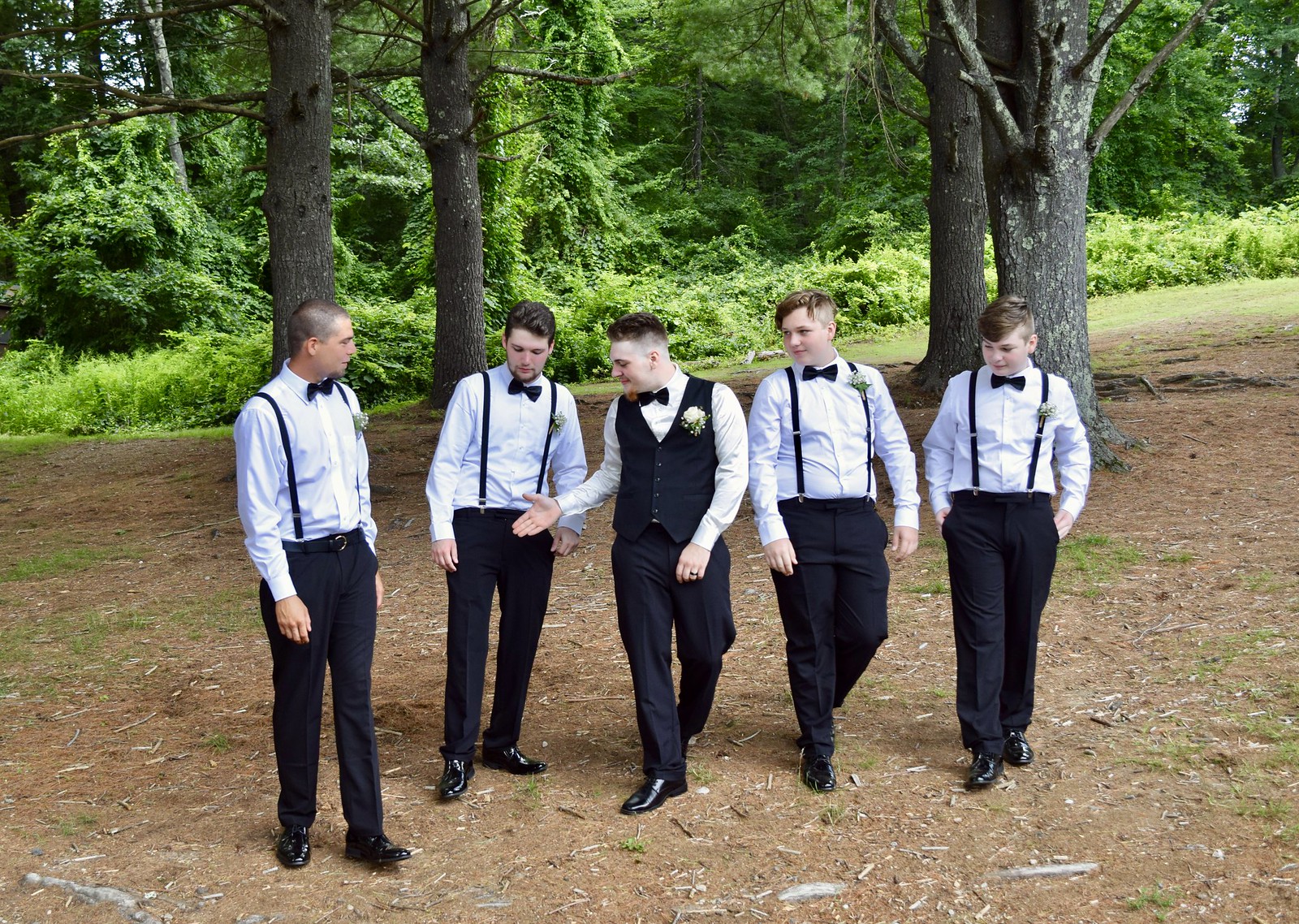This image captures a group of five young Caucasian males, likely in their late teens, standing together on bare dirt with some woodchips and small tree roots scattered across the ground. Surrounding them are patches of grass, ferns, and several trees, contributing to the lush greenery in the background, which even includes a large swath of kudzu plant. The focal point of the group is the central figure, who appears to be a groom, dressed in a classic wedding outfit consisting of a white shirt, black bowtie, black vest, black pants, and shiny black dress shoes. He is extending his hand for a handshake, revealing a ring on his ring finger and a boutonniere featuring a white flower on his left side. This man has short brown hair and a red goatee with shaved sides. Flanking him are four men, each wearing similar attire: white collared shirts, black bowties, black pants, and black dress shoes, differentiated only by their black suspenders instead of vests. Each of these men also sports a boutonniere. The men have light peach-colored skin, short brown hair, and some facial hair—including beards and goatees. They are positioned in a relaxed, semi-casual stance, indicative of a special occasion, likely a wedding, despite their youthful appearance.